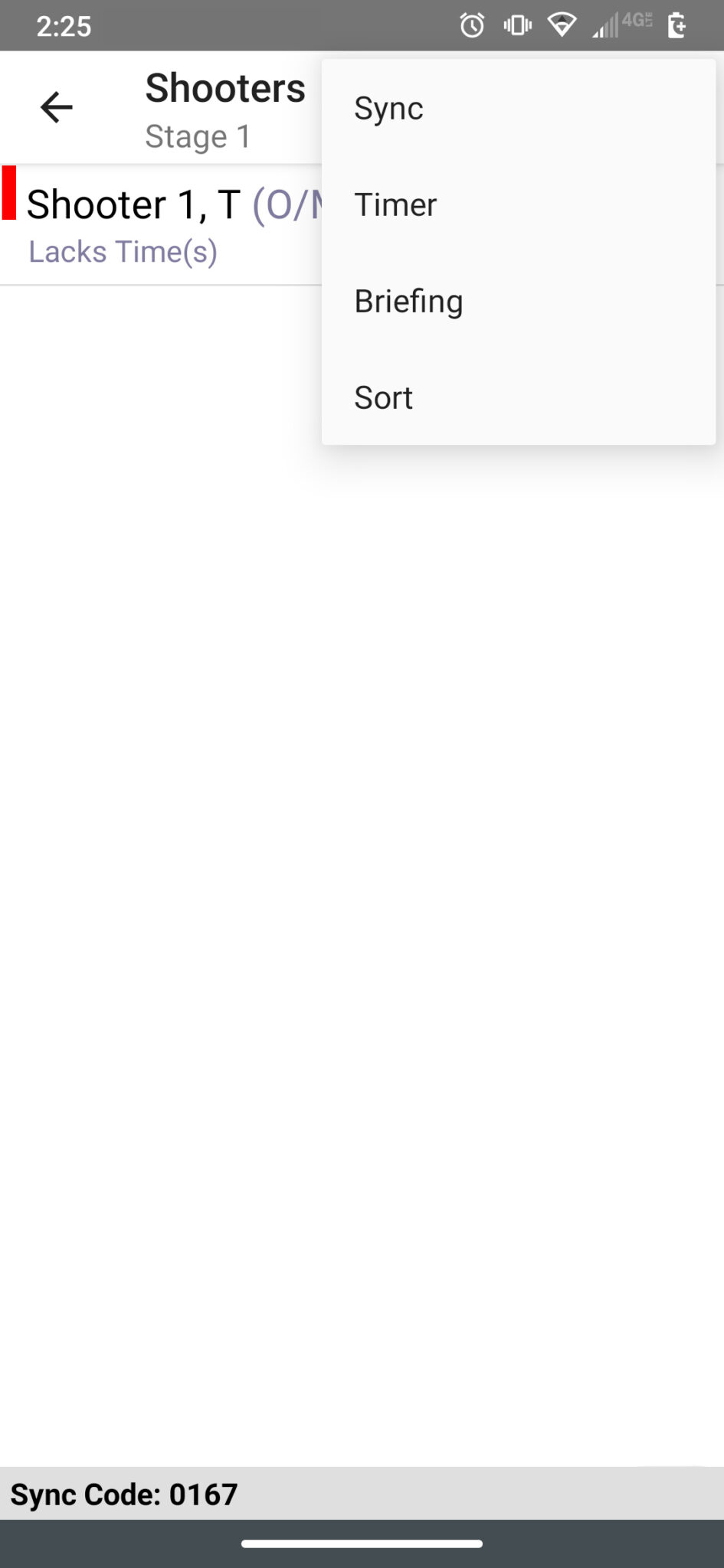The image appears to be a screenshot taken from a smartphone, capturing an app interface. The top section features a gray status bar displaying the number "225" on the upper left corner. Moving to the right, there is a clock, followed by a rectangle with vertical lines on its sides. Next to it, the Wi-Fi signal indicator is visible, followed by cellular signal bars indicating "4G LTE." The battery icon has a small plus sign on top of it.

Just below this status bar, in the upper left-hand area, the word "Shooters" is displayed in bold black letters. Directly beneath it, in gray font, it says "Stage One," accompanied by a right-pointing arrow. Progressing further down, there is a small red bar, adjacent to which it reads "Shooter 1, T" with "0/" partially visible due to a blocking box. This text also includes the phrase "lax times." 

To the right of this, there is a vertical box listing four words: "Sync," "Timer," "Briefing," and "Sort." At the bottom of the screen, a sync code "0167" is displayed above a light gray line, and beneath that is a dark gray rectangular area.